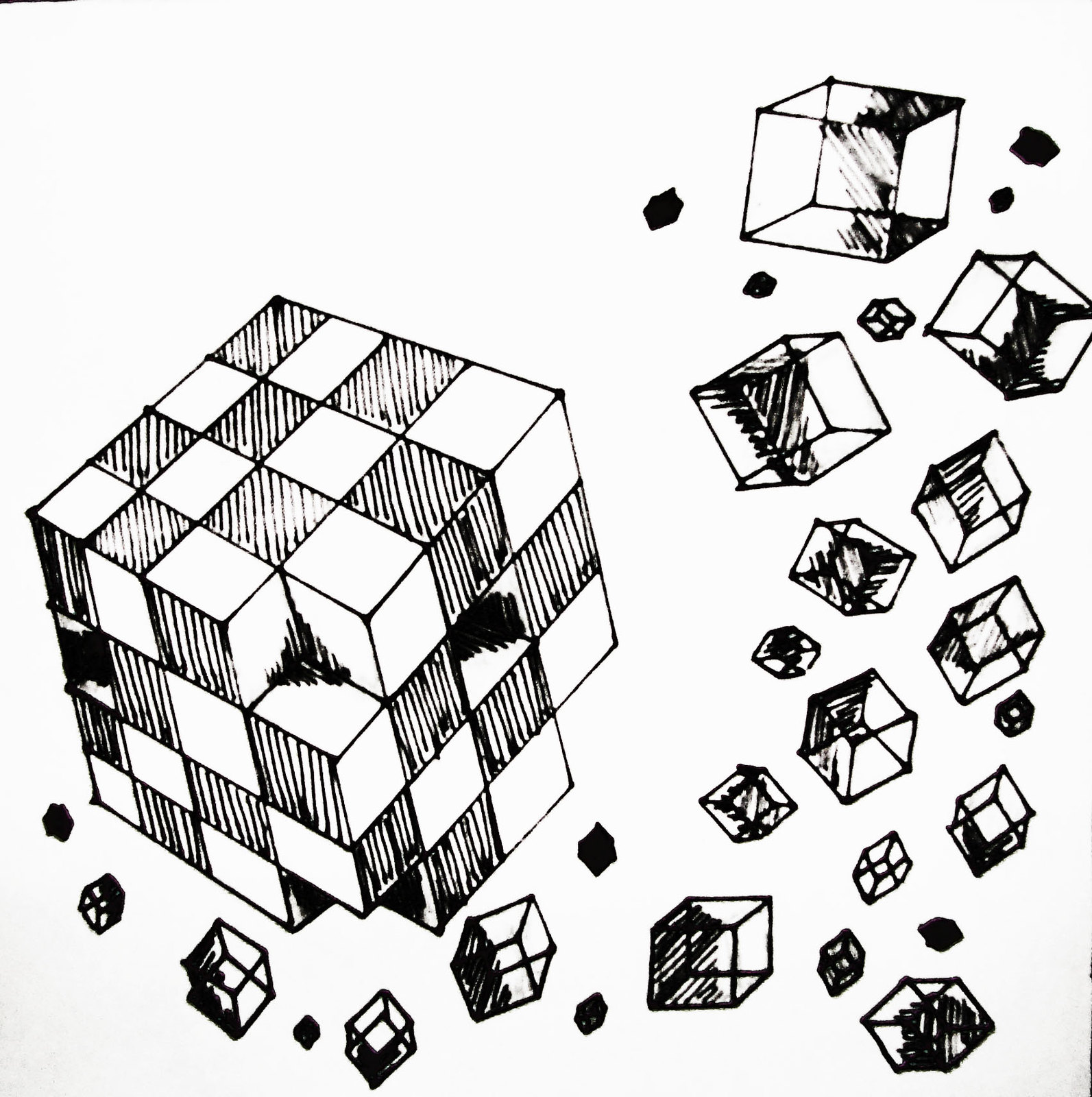The image is a detailed black-and-white drawing featuring a large 3D cube constructed from smaller cubes, positioned toward the left side of the composition. This large cube exhibits a checkered pattern with alternating squares shaded in black and white. Many black squares display diagonal striping, while the white squares remain plain. The cube is tilted, allowing a view of its top and two sides, with several pieces missing around its edges—particularly in the bottom middle, bottom right, and top front corners, creating visible gaps filled with stippled shading.

Surrounding the large, detailed cube are several smaller cubes dispersed primarily towards the right and bottom sections of the image, which might represent the missing pieces from the central structure. These smaller cubes vary in size, decreasing as they drift outward, contributing to a sense of motion as if they are floating away into the sky. The background remains plain white, emphasizing the stark contrast and abstract nature of the cube-centric design.